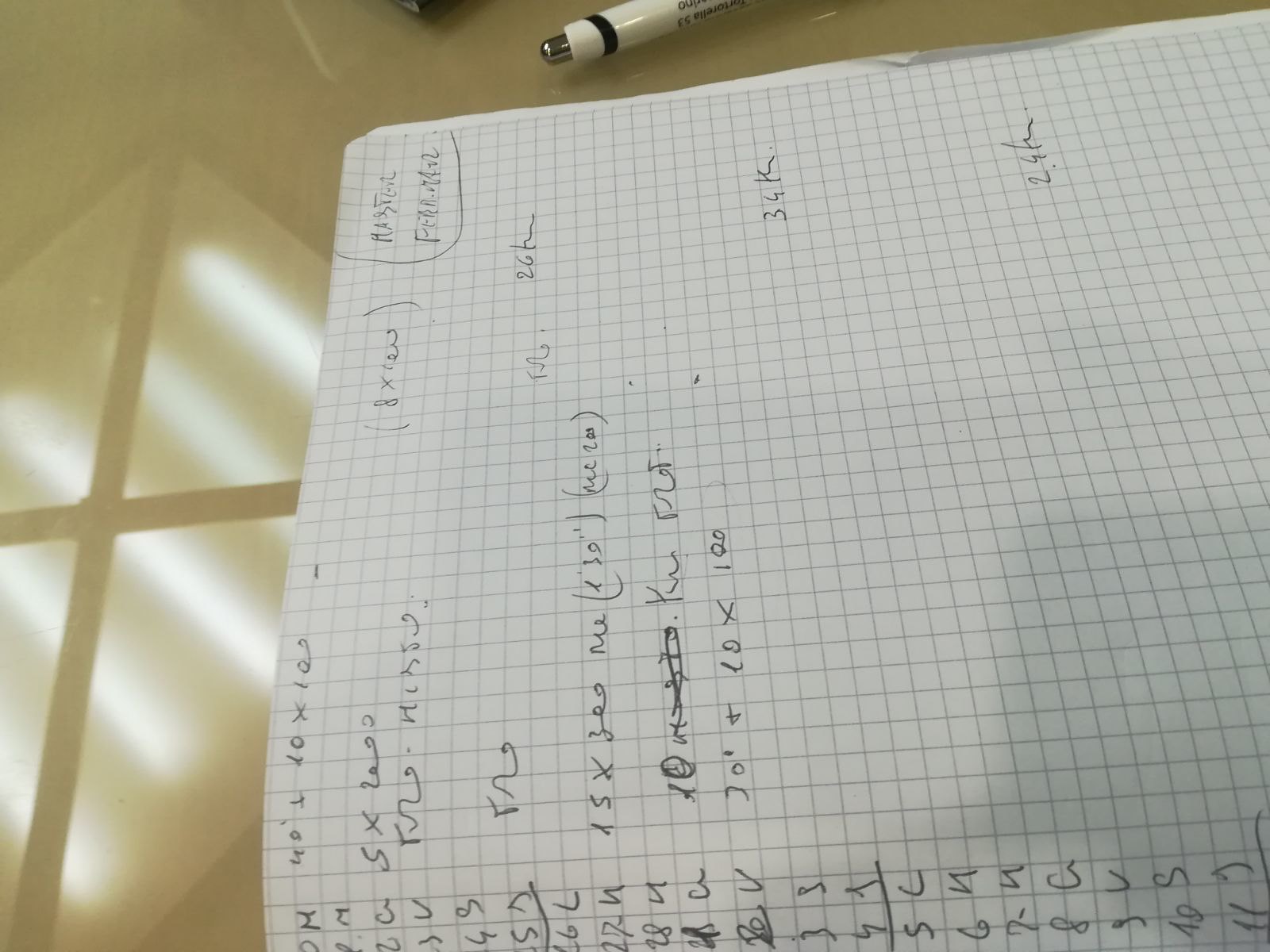This photograph captures a piece of graph paper positioned perpendicularly to the camera, causing the writing on it to appear sideways. Down the left-hand side of the paper, there are numbers written in a somewhat tidy but not very neat script. It starts with the numbers one through five, although the exact sequence might be interrupted due to the handwriting's style. The numbers appear in three distinct sections. The first section contains about six numbers, the second section consists of seven numbers, and the third mirrors the second with seven numbers as well. Each number is followed by a capital letter, including M, V, S, L, and U, although deciphering the exact letters is challenging due to the handwriting.

Under each sequence of numbers, there is a horizontal line separating the sections. Additionally, some equations are written on the page, though they are hardly legible; an example includes something resembling "30 + 10 * 100." The surrounding context reveals part of a tabletop, indicated by a reflection of light on its surface. The graph paper sits directly on this table, providing a workspace feel to the image.